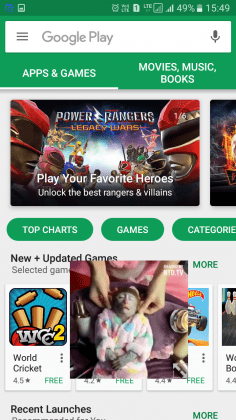This image is a screenshot of an antiquated version of the Google Play app. Dominating the top portion of the interface is a simple, white search bar labeled "Google Play." Below it, the screen is populated with a variety of downloadable games and apps. The first prominent game displayed is "Power Rangers: Legacy Wars." Further down, navigation options include "Top charts," "Games," and "Categories." Among the showcased applications are titles like “World Cricket” and a Hot Wheels racing game. Centered at the bottom of the screen, there is an intriguing image of a person's hands resting on the head of an animal, which appears to be a monkey. The monkey, dressed in a light pink robe, has its eyes closed and is reclining on a purple blanket. The overall design of this old Google Play layout features a predominantly white and green color scheme. In the upper right-hand corner, a digital 24-hour clock displays the time as 15:49.